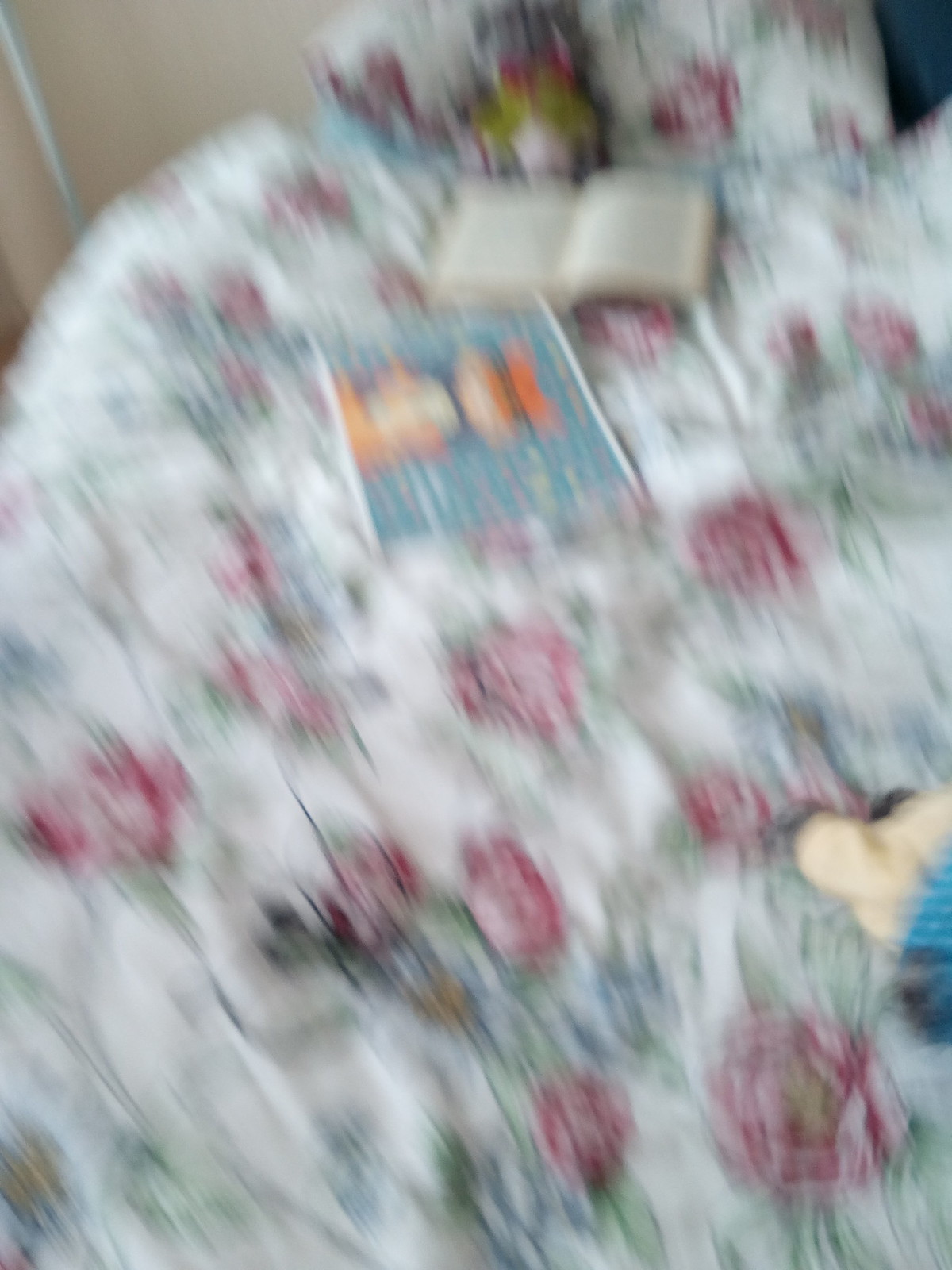In this somewhat blurry photograph, a neatly spread comforter adorns a bed. The comforter features a delicate floral pattern with green stems and leaves, accented by pink blossoms. Resting on the comforter, two books are visible. One is a brightly colored children's book, depicting what seems to be a fox dressed in a white and blue shirt. The other book lies open, displaying indistinct, grayish text on its tan pages. In the background, a tan wall is partially visible, accented by a silver stripe, likely indicating the presence of a floor lamp. The overall scene evokes a sense of quiet, cozy leisure.